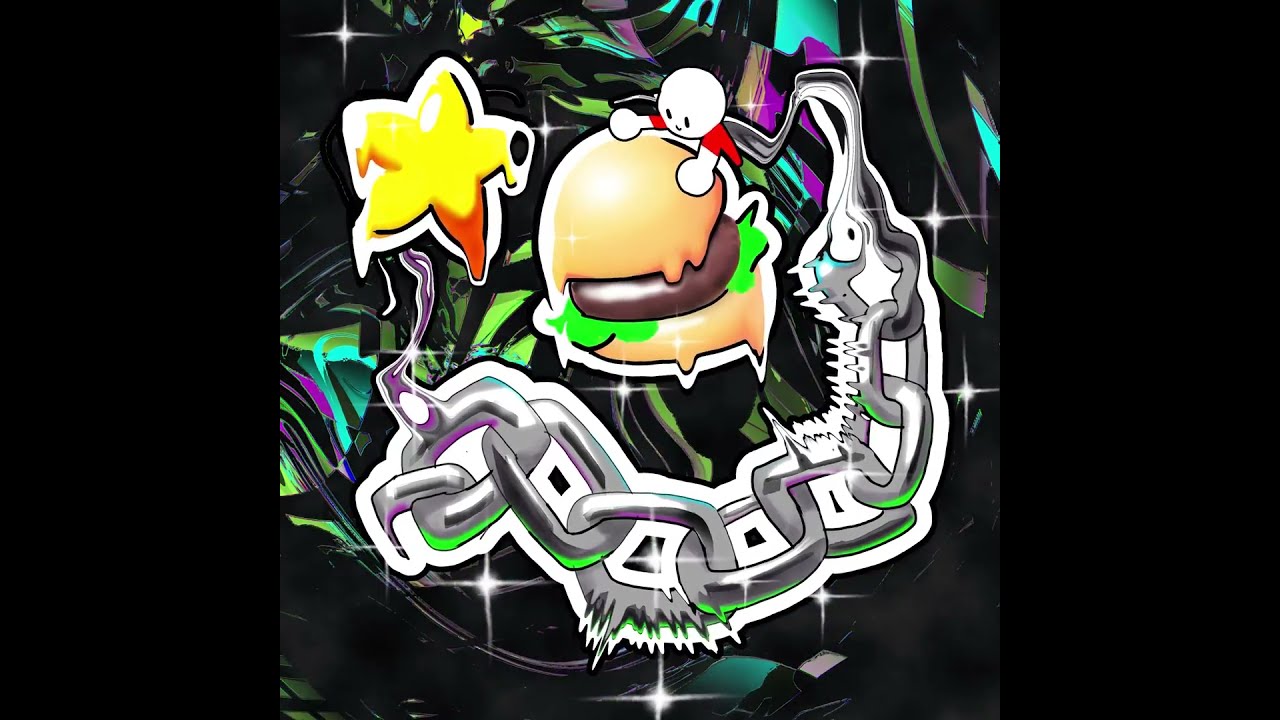The image is a vibrant and intricate graphical design with a distinctive graffiti style, bordered on both the left and right by solid black rectangles, each occupying roughly 20% of the image's width. In the center, there's a colorful assembly featuring a hamburger with a beige bun, a brown patty, and vivid green lettuce. Atop the hamburger, a small white figure with a bubble-shaped head and circular hands, dressed in a red shirt, leans forward with a smile, as if embracing the bun. To the left of the hamburger floats a yellow star with five points, four of which appear to be melting downwards and are outlined in white. This star features one red point among the yellow ones.

Beneath and coiling around the hamburger and star is a silver chain. The chain, some sections of which are jagged and fuzzy as if reacting to an unseen force, loops around and connects to the back of the white bubble character. The background of the middle panel is a dynamic swirl of greens, blues, and purples, reminiscent of an oil painting, infused with varying hues and twinkling stars that add to the image's otherworldly aesthetic.